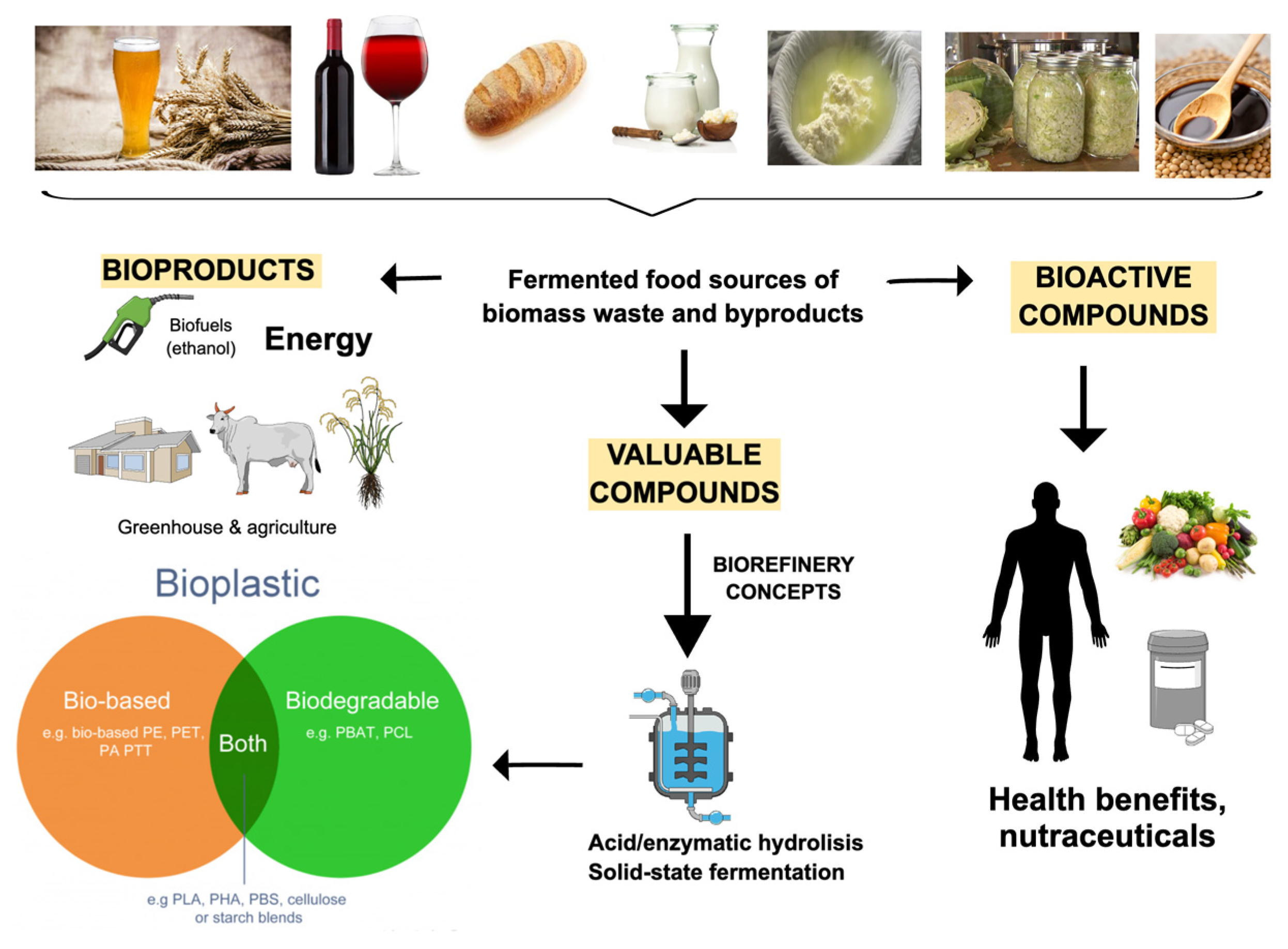The image features a comprehensive diagram on a white background without visible borders, titled "Fermented Food Sources of Biomass Waste and Byproducts." At the top left of the image, there is a photograph of a pint of beer with yellow liquid and white foam, positioned next to a pile of hops. To the right, a black bottle with a red cap is accompanied by a glass of red wine. Continuing to the right, there is a yellow baguette and then two bottles of white liquid, possibly milk or cream, with the smaller bottle in front. Further right, the image transitions to a bucket containing what may be curdled cheese, followed by bottled cabbage and, on the far right, a bowl of sauce atop some beans.

Below this row of images, a horizontal line leads to black print in the center that reads "Fermented Food Sources of Biomass Waste and Byproducts," flanked by arrows pointing both left and right. The left side features arrows labeled "bioproducts," "biofuels," "energy," and "greenhouse agriculture," accompanied by images of a gas pump handle, a plant, and a cow or bull in a house. In the center, an arrow points to "valuable compounds," leading to text about "biorefinery concepts," "acid enzymatic hydrolysis," and "solid-state fermentation." A leftward arrow indicates "bioplastic" with two overlapping circles labeled "biobased" and "biodegradable." To the right, "bioactive compounds" is connected by an arrow pointing down to a human figure's shadow, fruits, and medication, highlighting "health benefits" and "nutraceuticals."